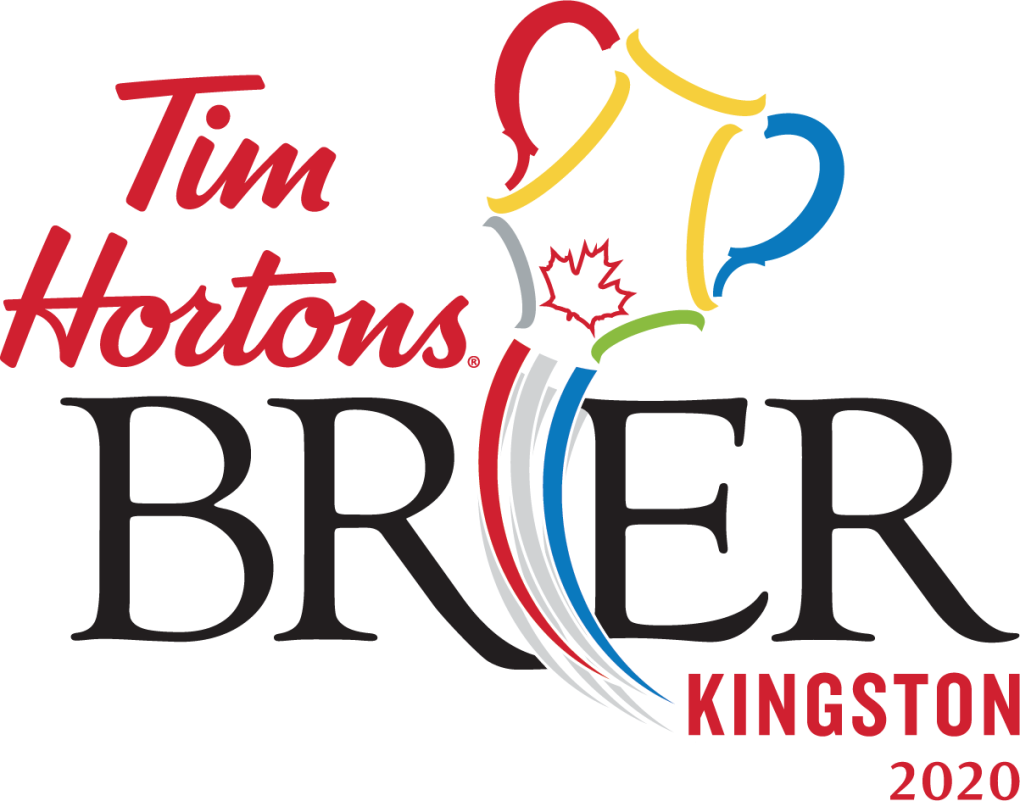The image showcases a promotional design on a plain white background with no visible borders. Dominating the upper left corner, "Tim Hortons" is written in elegant red cursive, occupying approximately 25% of the space, with a registered trademark symbol (®) beside it. Below this, in bold black letters stretching from left to right, is the text "B-R-E-R." Intersecting the gap between the letters 'R' and 'E' is an elaborately artistic trophy. 

The trophy features a multicolored theme: the left handle is red, the right handle is blue, the top half has gold outlines, while the left side of the base is silver or gray and the right side is green. Centered within the trophy's design is a white maple leaf outlined in red. Further enhancing the visual complexity, three lines—one red, one silver, and one blue—swoosh upward between the R and the E towards the trophy. Additionally, anchoring the lower right part of the image, beneath the 'E-R,' the text "Kingston 2020" is displayed in bold red print.